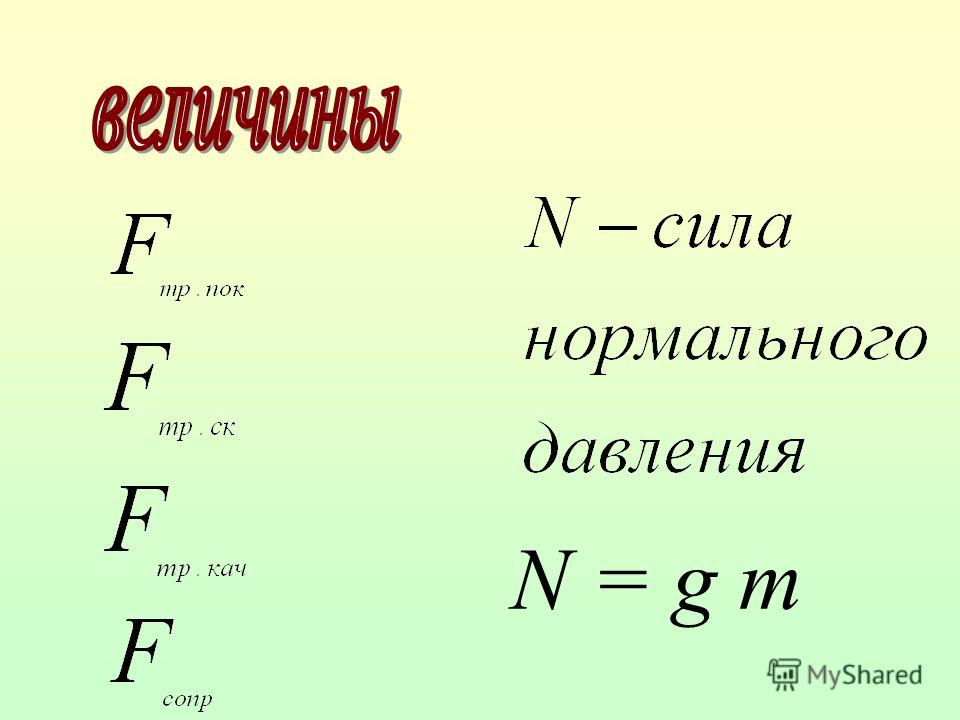This color infographic features a landscape orientation and employs a soft gradient background transitioning from pale green at the bottom to light yellow at the top. The backdrop is composed of light pastel shades. The primary content of the graphic is text in what appears to be the Russian language, which is prominently highlighted in various fonts and colors.

In the upper left corner, a bold red, slightly italicized word in Cyrillic letters reads "B E" followed by various other Cyrillic characters (possibly spelling "BEHUUBL"). Below this, there is a vertical column of four capital "F" letters, each italicized and in a bold serif font, with accompanying small Cyrillic footnotes next to them.

On the right side of the infographic, a column of scientific notations is displayed. The first line starts with the letters "N-C-U" followed by Cyrillic characters "P-A". Below this, two long words in Russian are written. The bottom-most equation on this side reads "N = G M". 

In the very bottom right corner, there is a minimalistic black line art icon that resembles a bar graph, followed by the text "my shared" in black.

This infographic combines elements of illustration and graphic design with foreign language typography, effectively conveying scientific information through its detailed and structured layout.